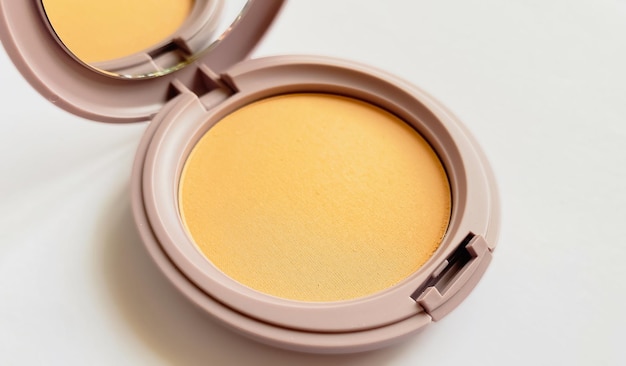The image captures an open makeup compact resting on a white surface, revealing both its contents and structure. The compact, shaped like a small round clamshell, features a hinged lid and a latch mechanism. The exterior of the compact is made from plastic, showcased in a blend of beige and a pinkish-lavender hue. On the inside of the lid, a small mirror is visible, reflecting the makeup housed in the bottom part, which is a light orangish-brown or creamy orange shade, reminiscent of pressed powder or blush. Notably, the compact is missing its applicator pad, which is typically used for applying the makeup. The background is a very pale blue-gray, contrasting subtly with the compact's colors. The setup appears neat and unused, with no visible signs of prior use on the makeup surface.